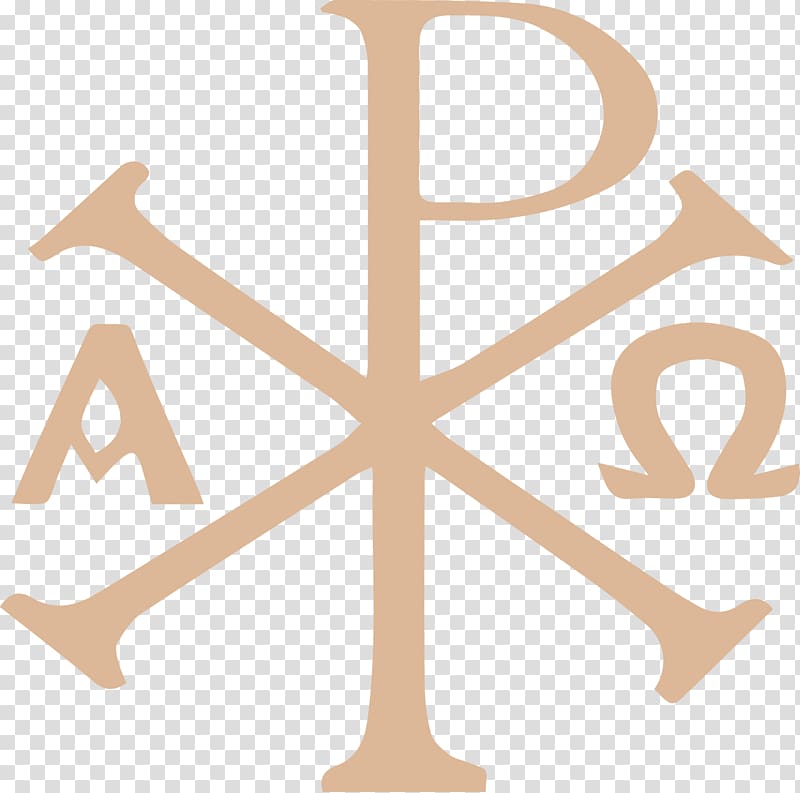The image features a centrally positioned dark tan symbol on a grey and white checkered background, indicative of a transparent image. The core of the symbol is dominated by a long, vertical letter 'P' which extends from the top to the bottom, creating a six-spoke design reminiscent of an asterisk or a cross. This 'P' intersects with the cross shape, with two short horizontal lines protruding from each side of the vertical 'P'. To the left of this assembly is the Greek letter 'Alpha (A)' and to the right is the Greek letter 'Omega (Ω)', forming a symmetrical arrangement. The plain checkered background underscores the symbol, emphasizing the central design intended for easy copying and pasting into other documents.